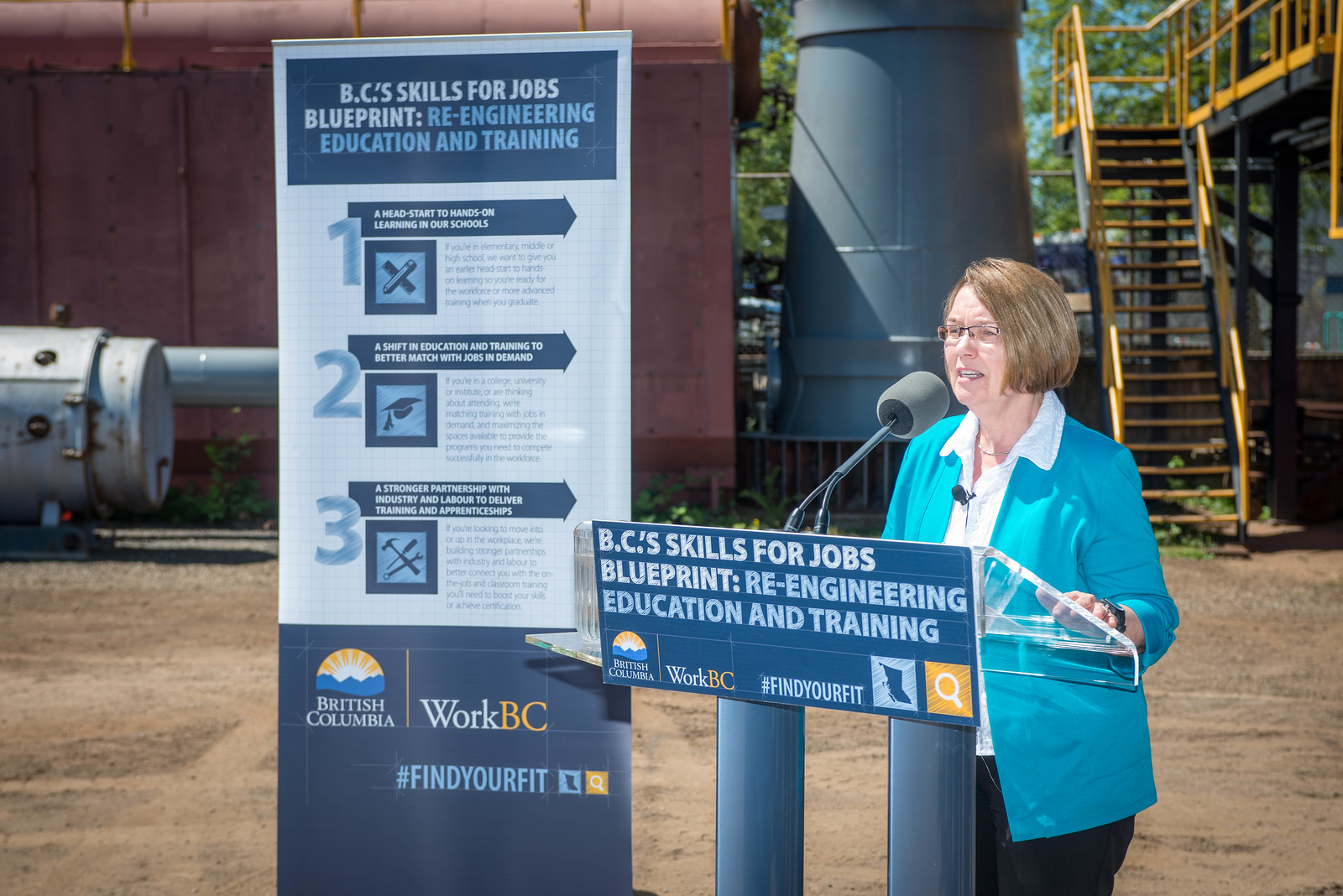This horizontally aligned, landscape-oriented color photograph captures a woman speaking at an outdoor podium. The podium in front of her features two blue legs and a prominently displayed blue sign. The sign bears the text "BC's Skills for Jobs Blueprint: Re-engineering Education and Training" in white and light blue lettering. The lower left corner of the sign contains the British Columbia logo, and beside it, the text "WorkBC" and the hashtag "#findyourfit." 

The woman standing behind the podium is leaning on a clear plastic piece and is dressed in a light blue suit jacket over a collared white button-down shirt. She has short brown hair, wears small wire-rimmed glasses, and has a microphone clipped to her shirt, while she speaks into a large gray microphone. Her mouth is open, indicating she is mid-speech, and she appears to be in her 50s. 

To the left of her and the podium, there is a vertical banner with the same heading as on the podium, alongside a bulleted list of three policy points that are too small to read clearly. The ground she stands on is dirt, and the background reveals an industrial setting, including a cylindrical gray building, an old and rusted red sheet metal building, and yellow metal stairs leading up to a platform. The ambiance suggests a location such as a construction site or industrial park.